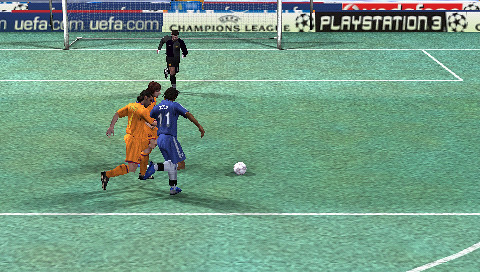The image captures a somewhat grainy, vintage screenshot from a soccer video game, likely from the FIFA series, given its small and compressed format. The aspect ratio of the image appears notably wider than it is tall, with dimensions roughly two and a half times its height. Central to the scene are four players clustered just inside the goal box on a green soccer field marked with white lines.

In the foreground, a player wearing a blue jersey, numbered 11, is prominently dribbling the ball, his posture suggesting forward movement with his foot held back, poised to kick. He is closely contested by two defenders in orange jerseys, who are running towards the ball, their focus intently on intercepting the attack. All three players are facing generally in the same direction, towards the right side of the image.

Further in the background, near the goal situated at the center-left of the scene, a fourth figure is present. This player appears to be the goalkeeper, attired in what appears to be either a black or very dark blue outfit, captured in mid-run, likely preparing to defend against the impending shot.

The backdrop also features various advertisements, lending an authentic feel to the gaming environment. Visible banners include the UEFA Champions League, uefa.com, and PlayStation 3, further dating the image and solidifying its context within a past era of gaming. These elements combine to create a dynamic portrayal of an in-game moment, filled with action and anticipation.